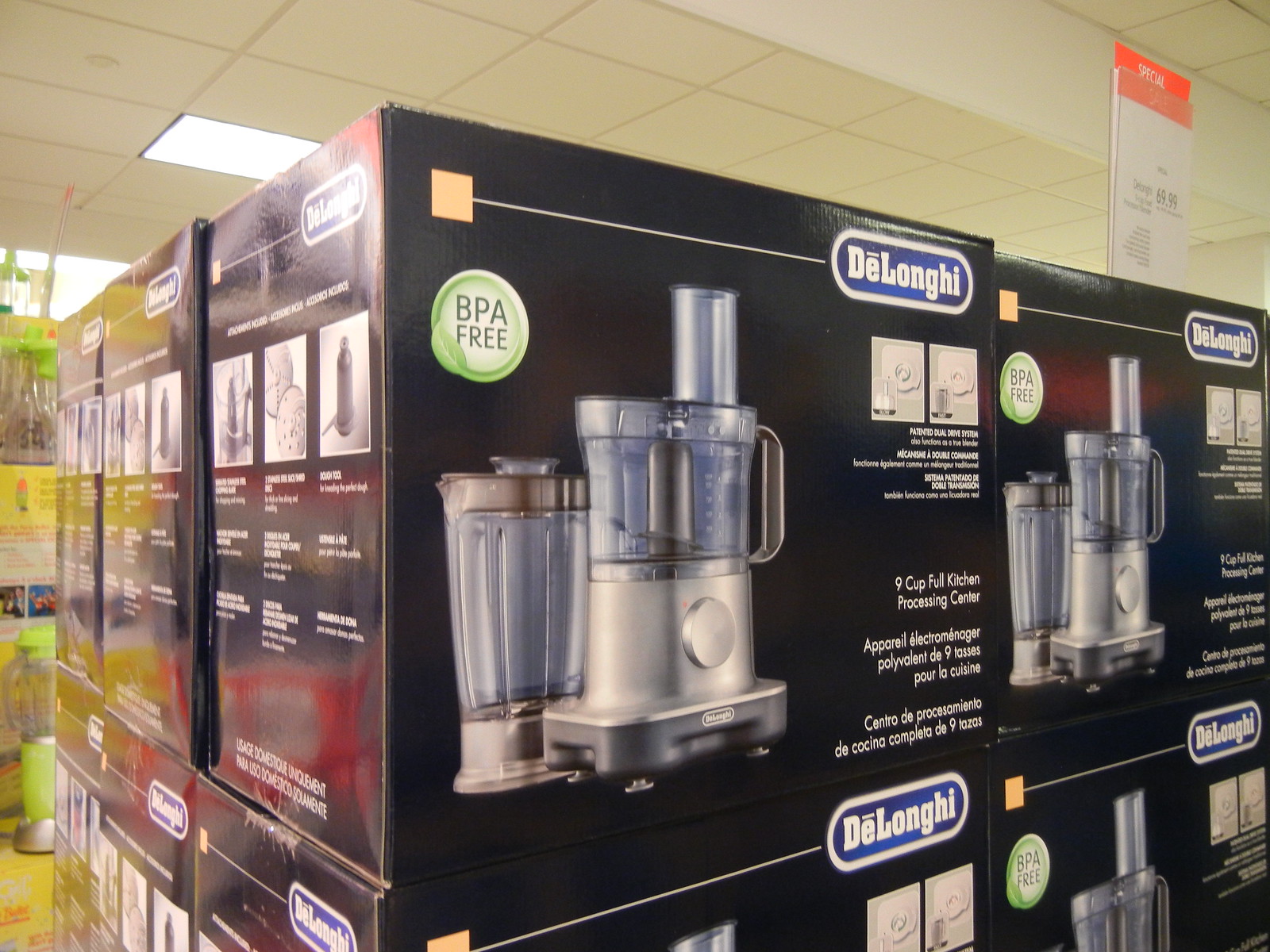This color photograph captures a neatly stacked display of DeLonghi food processor boxes in a big box store, possibly Walmart or Target. Each black cardboard box prominently features the DeLonghi brand name at the top. The front of the box displays a vivid image of the food processor, highlighting its signature top pipe for food insertion. Adjacent to this, another attachment resembling a blender is shown. Text on the box emphasizes key features, including "BPA Free," "Patented Dual Drive System," and "9 Cup Full Kitchen Processing Center," which are also translated into French and Spanish. Additionally, a green leaf icon reinforces the BPA-free claim. The stacked arrangement suggests a promotional display without any presence of people, animals, or buildings in the frame.